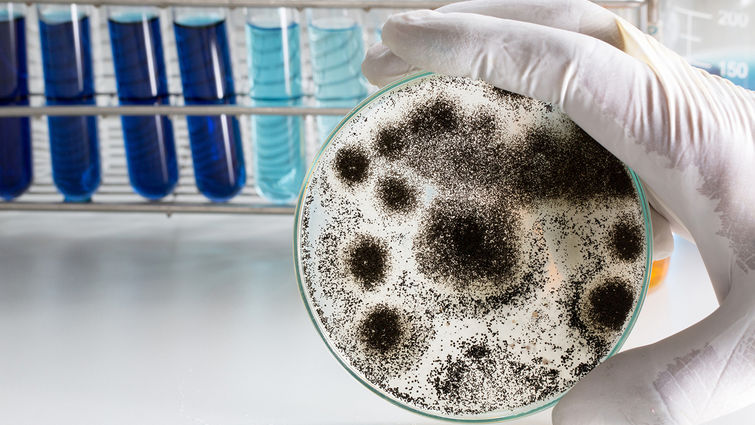A gloved hand is prominently holding up a petri dish, showcasing a diverse array of black spots against a white background, possibly indicative of mold or fungus growth. The dish features a mixture of small to large black spots, with some forming distinct diagonal patterns. Specifically, there is a large black circle near the center, surrounded by smaller dots at various positions, including a notable cluster at the ten o'clock position and another at four o'clock. The hand, clad in snug white gloves, is positioned against a scientific workspace. In the background, a white table supports a tray of test tubes. This tray, situated on the left side of the image, contains four test tubes filled with dark blue liquid and three others with light blue fluid. Additionally, a beaker marked up to 150 milliliters and filled with light blue liquid is visible to the right, adding to the scientific ambiance of the scene.